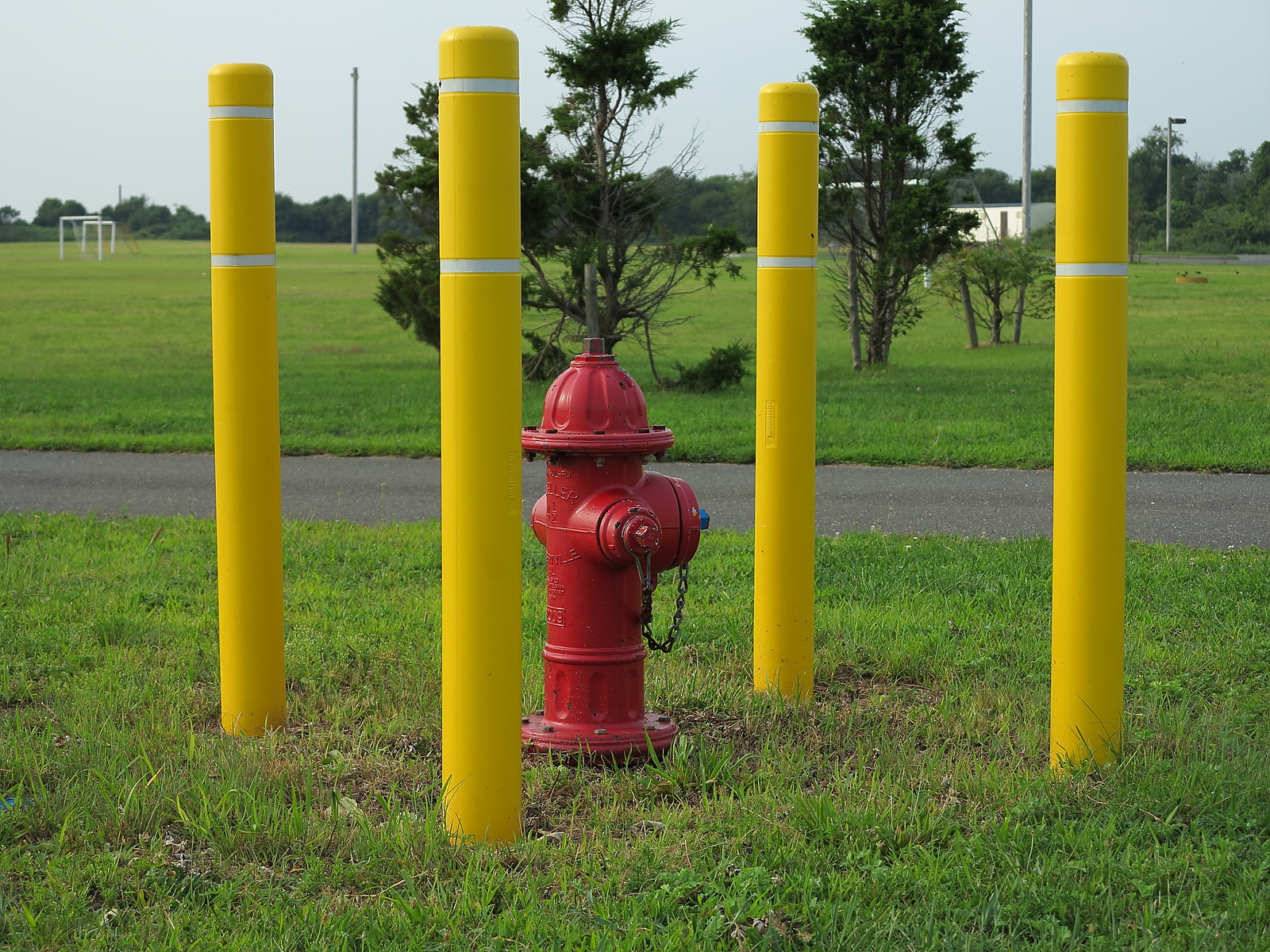This photograph, taken outdoors during the daytime, features a red fire hydrant surrounded by four bright yellow safety posts, each adorned with two white stripes near their tops. The posts, approximately twice the height of the hydrant, are firmly embedded in a green grassy area with some brown patches in the foreground. The scene is set in what appears to be a park or sports field. A gray, paved path runs horizontally across the middle of the image, separating the fire hydrant and posts from the background. Behind the path, there are two thin-trunked trees with green foliage. Further in the distance, to the left, a white soccer goalpost can be seen, indicating the presence of a sports field. Additional trees and possibly a white building are faintly visible along the horizon, beneath a slightly cloudy gray-blue sky.